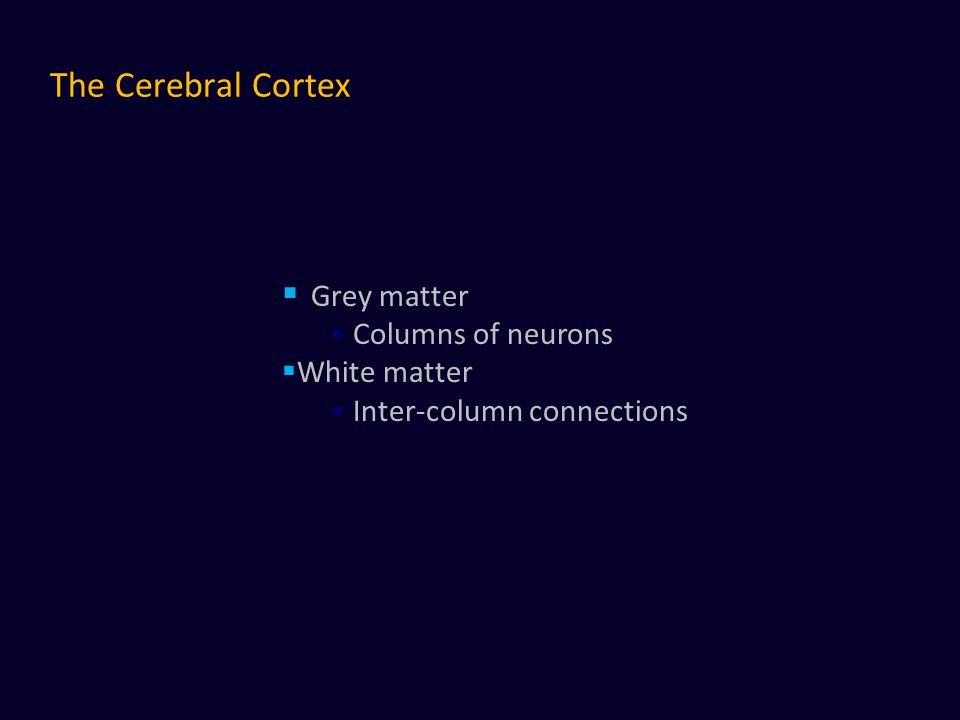The image appears to be part of a presentation slide with a dark blue background, featuring textual information predominantly in thin, yellow, and white fonts. In the upper left corner, the title "The Cerebral Cortex" is displayed in a yellowish text. Moving towards the middle, a light blue square bullet point precedes the term "Gray Matter." Adjacent to this, another dark blue rounded bullet point highlights "Columns of Neurons." Below these, following another light blue bullet point, the term "White Matter" is presented, and finally, another dark blue bullet point specifies "Inter-Column Connections." The slide seems to serve an educational purpose, explaining the structural and functional aspects of the cerebral cortex.